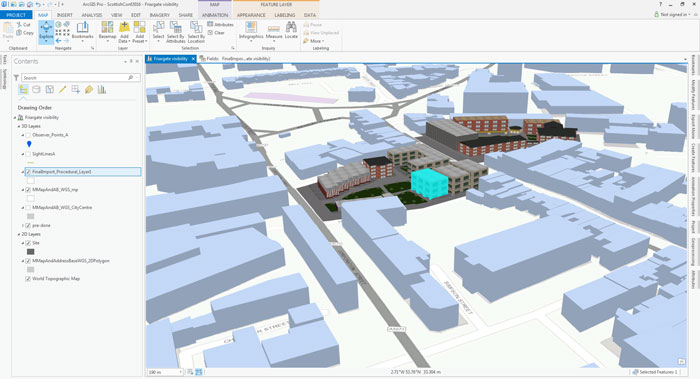The image showcases a detailed 3D model, likely created using CAD software, depicting a cityscape. The central area of the model features buildings with distinctive red facades and one prominent building painted bright blue, contrasting starkly against the predominantly gray, cubic structures surrounding them. These peripheral structures appear streamlined and modular. The streets are denoted by gray stripes, organizing the layout of the city. Notably, a highlighted section on one of the red buildings in the center is marked in turquoise, indicating active modification or focus within the CAD interface. The model includes various long buildings with numerous windows, and a bridge is visible at the upper part of the image, adding to the comprehensive urban detailing.